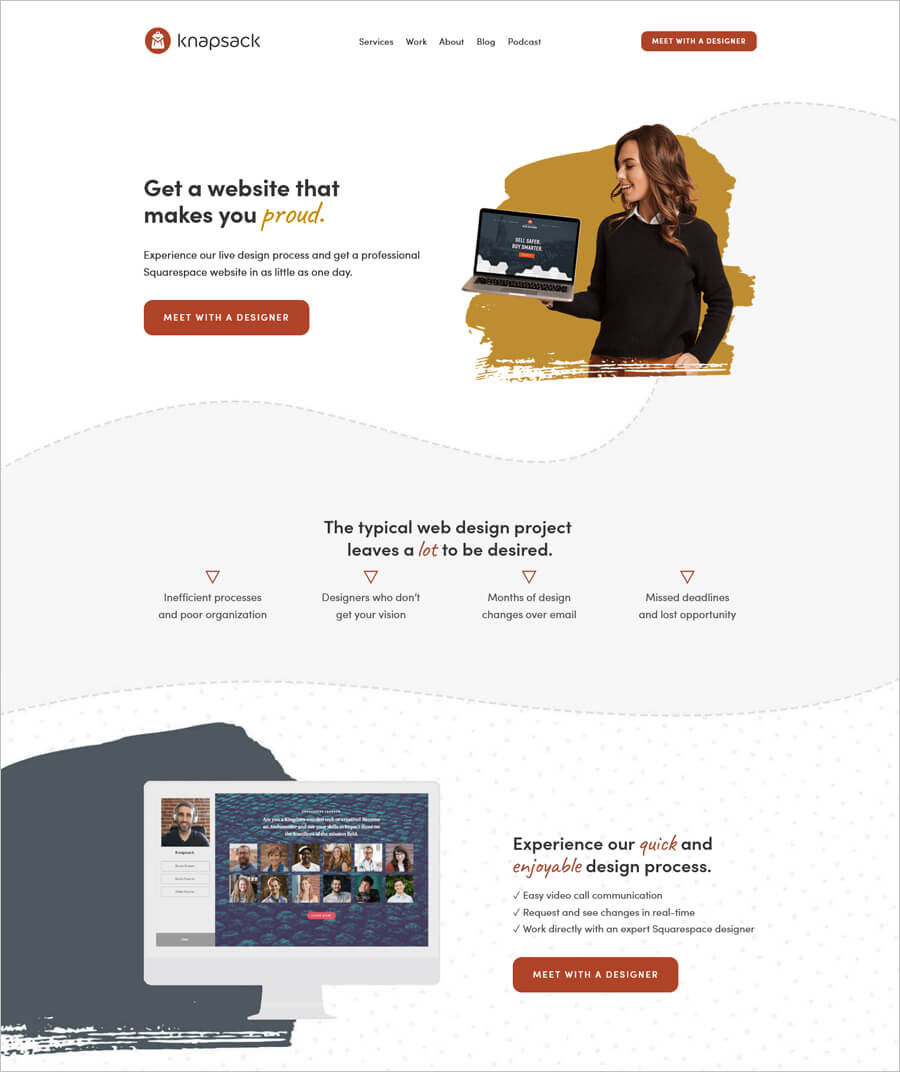On the web page for Knapsack, the top navigation bar features menu options for Services, Work, About, Blog, and Podcasts. The main headline reads, "Get a website that makes you proud." The site promotes their unique offering of a professional and personalized Squarespace website, promising completion in as little as one day through a live design process.

The page elaborates on the benefits of their service: "Experience our quick and enjoyable design process with easy video call communication. Request and see changes in real-time while working directly with an expert Squarespace designer." It contrasts this with the typical web design experience, which is often marred by inefficiency, poor organization, lengthy email chains for design changes, and missed deadlines.

Towards the bottom, the emphasis is on the streamlined experience: "Meet with a designer, and experience a seamless design journey." The final call to action encourages potential customers to engage with their efficient and client-focused design service.